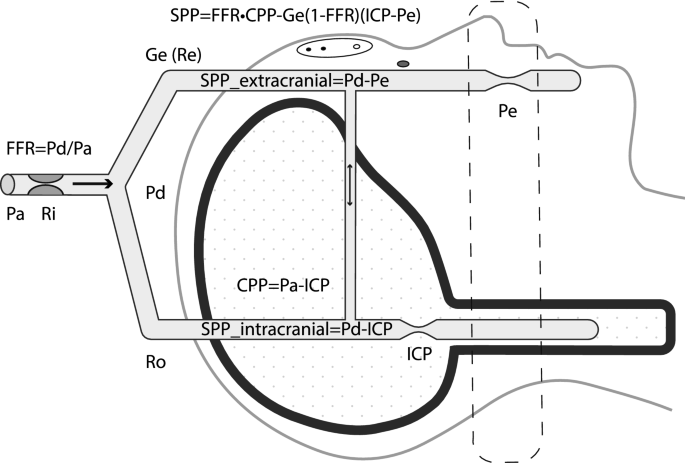This detailed illustration in black, white, and gray depicts a complex scientific diagram focused on the human cranium, likely used for medical or engineering purposes, such as planning brain surgery. At the top, the formula "SPP = FFR + CPP - GE (1 - FFR) ICP / PE" is prominently displayed. The diagram includes multiple labeled elements and pathways: one tube labeled "FFR PD / PA PA RI" branches into two paths marked "SPP extracranial PD PE" and "SPP intracranial PD / ICP." A prominent black circular line and vertical dotted lines frame and connect different parts of the illustration, indicating various scientific processes and connections within the head structure.